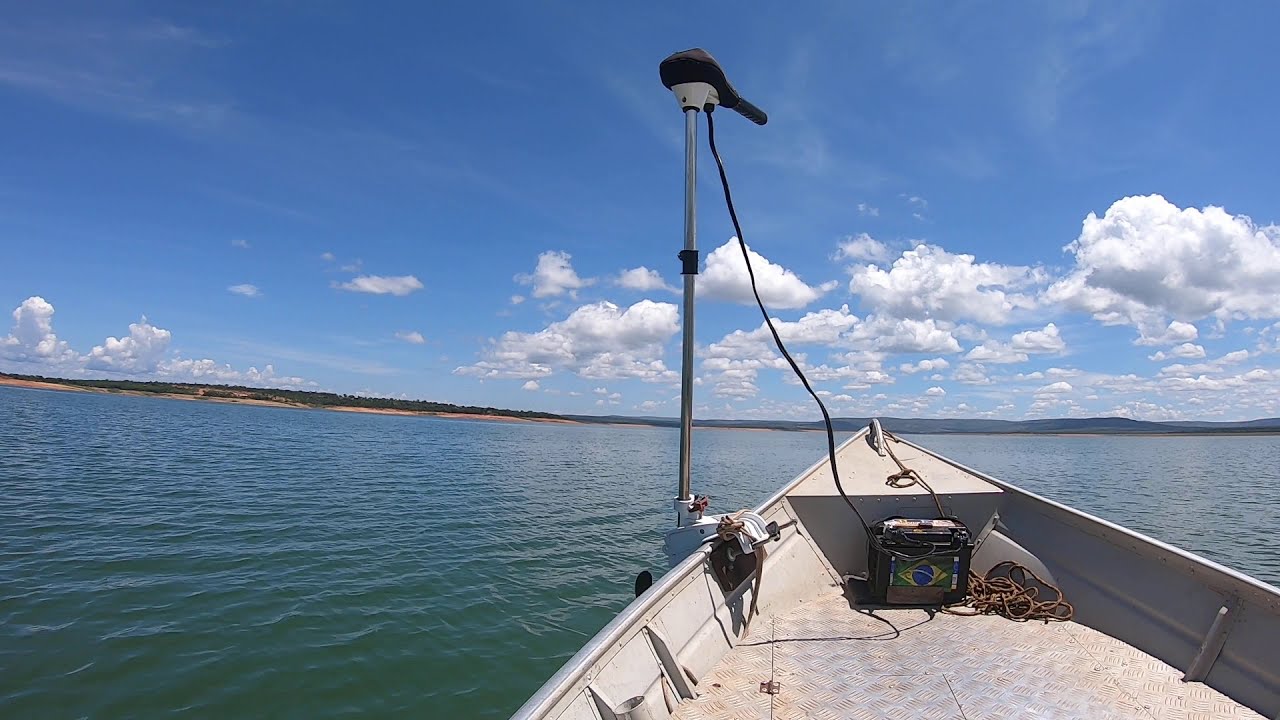The image depicts the front of a white boat, positioned in the bottom right corner, navigating through a large, greenish-blue body of water. The boat's deck features equipment, including a prominent black box connected to a long metal pole that extends vertically into the sky, with a silver shaft, a black top, and a gray bottom. A cord runs from this pole to the box on the deck. The water appears slightly wavy with subtle ripples. In the distance, a thin strip of land spans the horizon. On the left, the landmass resembles a beach with possible trees, while further out, it transitions to darker terrain with hills or mountains. Above, the sky is a clear, vibrant blue with clusters of small, puffy cumulus clouds floating primarily on the right and a few on the left, adding depth to the expansive view.